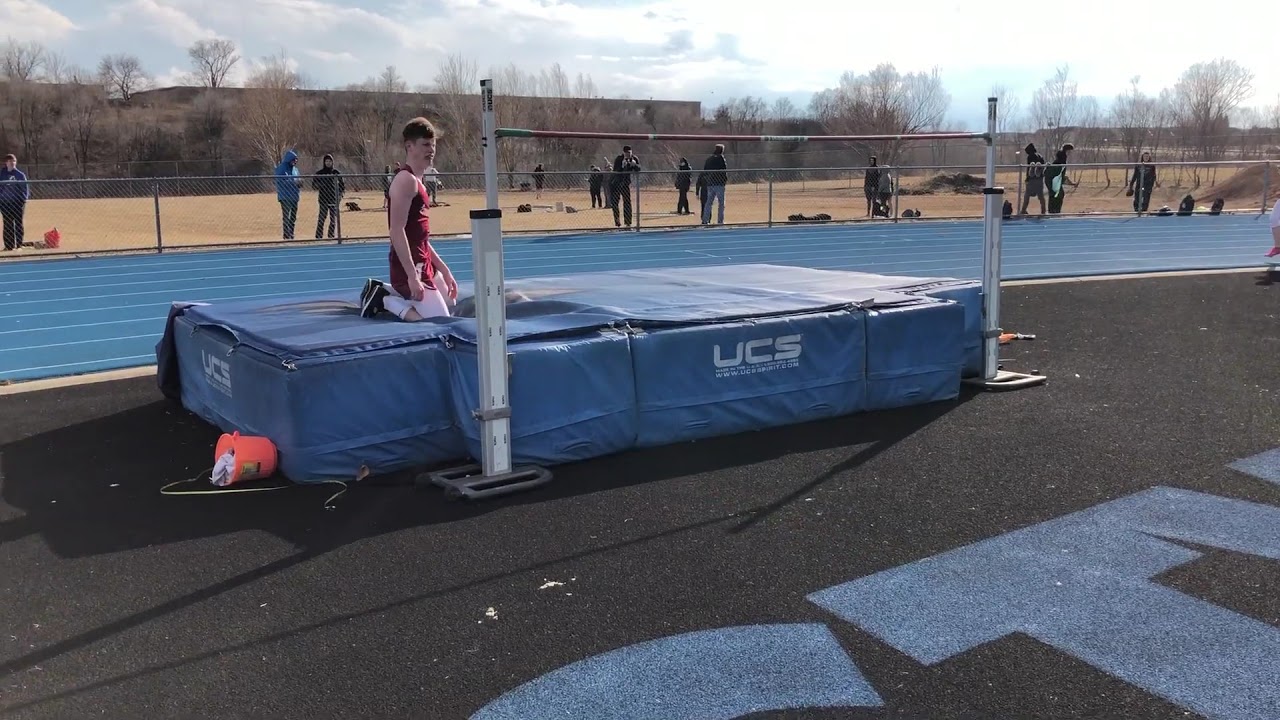In this detailed image taken at a track and field meet, a young male athlete, appearing to be around 16 years old, is captured on his knees on a large, thick blue safety mat after clearing a high jump. Sporting a dark red tank top with his school’s name starting with an "S," matching shorts, white socks, and black running shoes, he’s positioned near the center of the image under the red high jump bar supported by white vertical poles. The athlete is set against a backdrop of a blue running track with white lines, beyond which a gray fence separates the track from about ten spectators who are watching the event. The field behind the fence displays tan dead grass, and further back, a line of leafless brown trees is visible. Additionally, the mat features the branding "UCS" and the website "www.ucssprint.com," likely indicating the equipment's manufacturer.